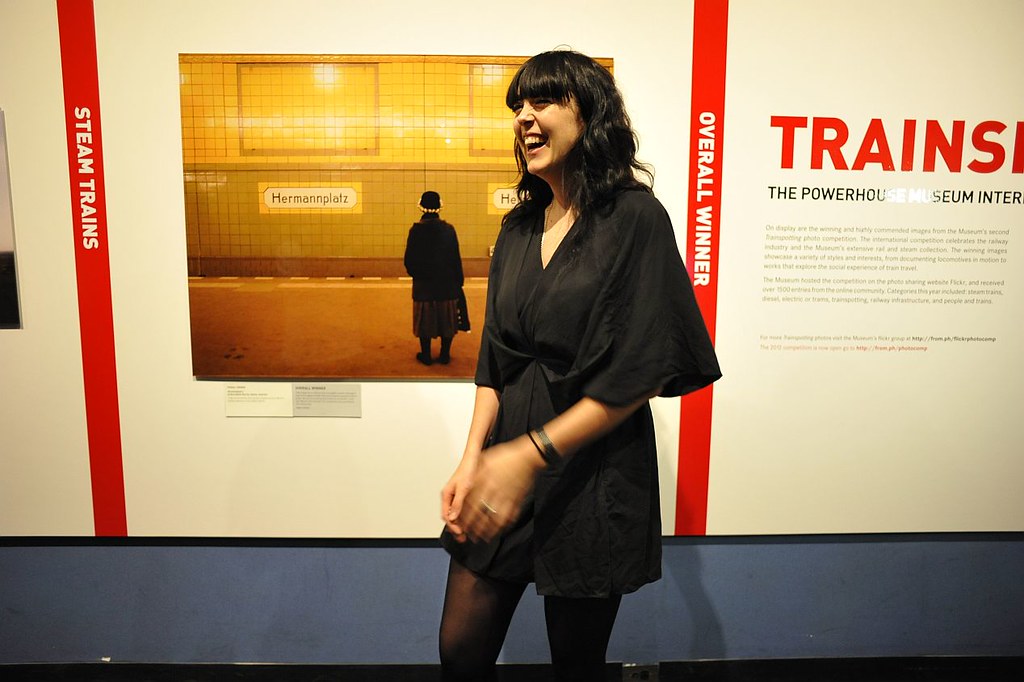In this photograph, a woman with shoulder-length, curly black hair and bangs is captured mid-laugh as she walks to the left. She is dressed in a black blouse with elbow-length sleeves, black skirt, black pantyhose, and a black bracelet on her left wrist. The background features a beige wall with red stripes running vertically, one labeled "Steam Trains" and the other "Overall Winner," both in white font. Additionally, there is a sign with red text reading "Trains" above "The Powerhouse Museum International" in black. She stands in front of a painted portrait depicting another woman, dressed in black peacoat, skirt, and hat, seemingly at a subway station named "Herman Platz." The floor of the room is dark blue, adding a contrasting element to the scene.